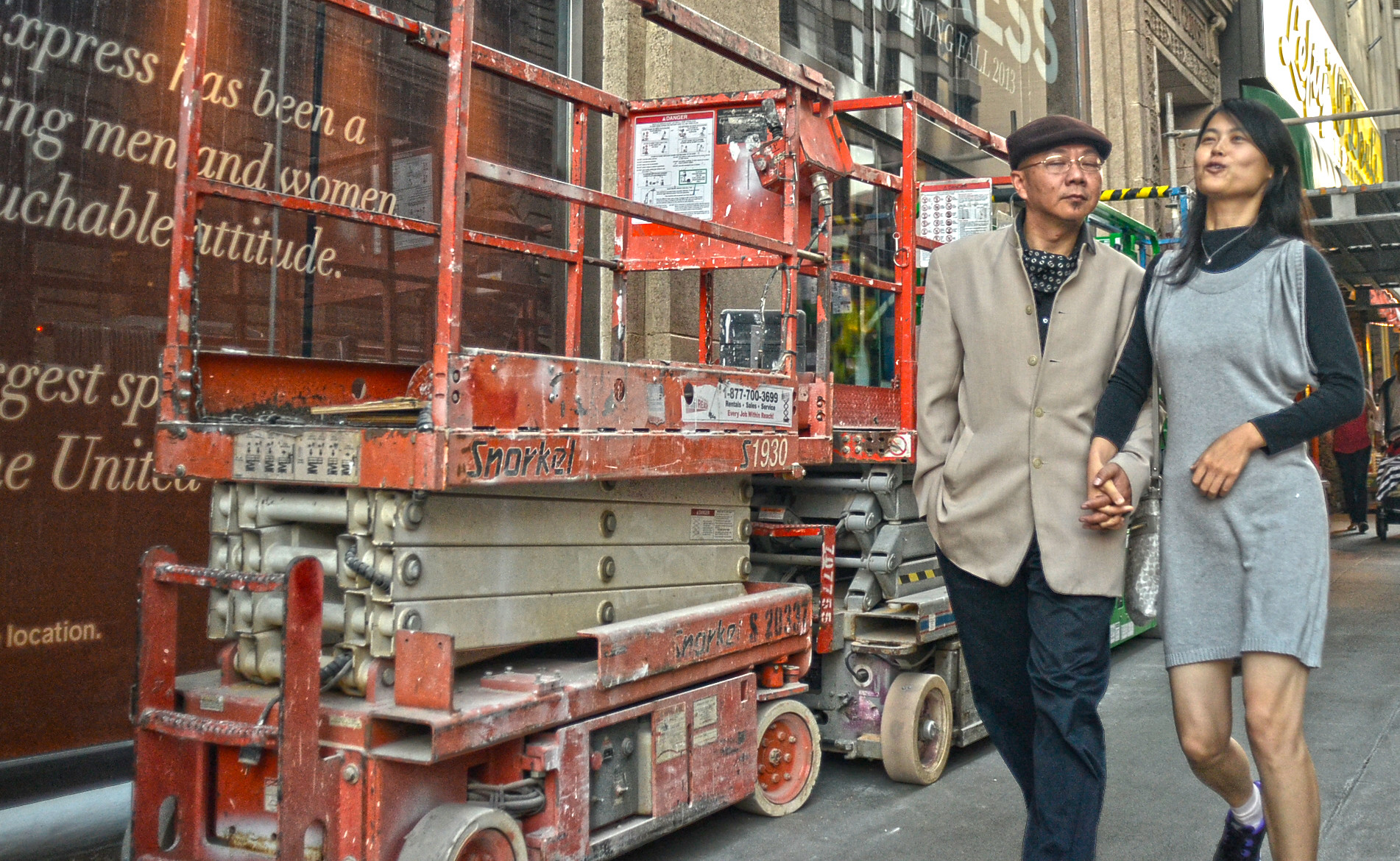In this daytime urban scene, a middle-aged Asian couple can be seen walking hand-in-hand on a city sidewalk. The man, dressed in black slacks, a tan overcoat, and wearing a brown flat cap along with wire glasses, is making playful faces at the woman beside him. The woman, donning a gray jumper dress over a black long-sleeve shirt, smiles warmly in response. Her dress ends just above her knees, revealing her legs. Both appear well-bundled, suggesting cool weather. To their left stands a red scissor lift, covered in dust and white paint, presumably for construction or window washing, with another silver lift visible behind it. Behind them, faded into the distance, are a few other pedestrians, while the surroundings feature buildings with unreadable signage indicative of a busy business district. This lively capture emphasizes the tender interaction between the couple amid their bustling, construction-adjacent surroundings.